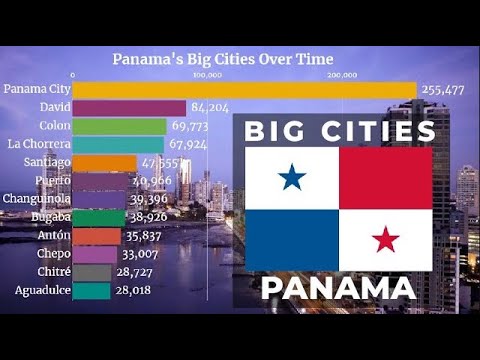This screenshot features a comprehensive depiction of Panama's major cities over time. The backdrop showcases a panoramic view of a coastline adorned with numerous boats, surrounded by towering skyscrapers and various business buildings, highlighting the city's dynamic architectural diversity. The central focus of the image is a collection of symbols and statistics: a prominent white rectangle with a vivid blue star sits opposite a striking red square, below which a white square with a red star and an adjacent blue square are displayed. This visual arrangement emphasizes "Big Cities, Panama."

The accompanying text provides population data for several key cities: Panama City boasts 255,000 inhabitants, David has 84,000, Colón houses 69,000, La Chorrera is home to 67,000, San Miguelito has 47,000, Las Tablas hosts 40,000, Changuinola has 39,000, Bugaba supports 38,000, Antón contains 35,000, Chepo is home to 33,000, Chitré shelters 28,000, and Penonomé has 28,000 residents. The juxtaposition of the thriving urban environment with these informative details paints a vivid picture of the evolving landscape and demographic distribution of Panama's big cities.